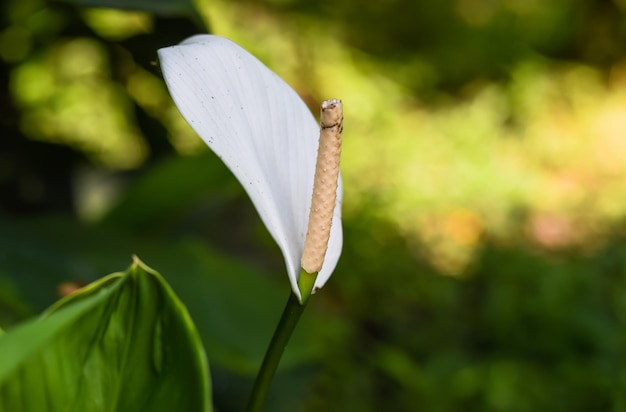The image is a close-up photograph of a single calla lily, prominently positioned toward the left side of the frame. In the foreground, there's a notable large green leaf located at the lower left corner, which partially obscures the base of the flower. The calla lily itself features one expansive, elegant white petal, which begins at a green base and transitions to beige as it extends outward. Near the tip of the petal, a distinct dark brown line encircles it, adding a subtle contrast. The middle of the flower showcases a slender, tube-like structure with a pinkish-brown hue, resembling a pine cone, which protrudes upwards. The stem of the flower is a darker green compared to the base of the petal. The background consists of blurry green foliage, likely other plants and leaves, which lacks specific details but suggests a lush, natural setting typical of an outdoor nature scene. Subtle light patches in the background may indicate sunlight filtering through the vegetation. This beautifully detailed image captures the intricate elegance of the calla lily, making it a lovely visual for enthusiasts of nature and botany.